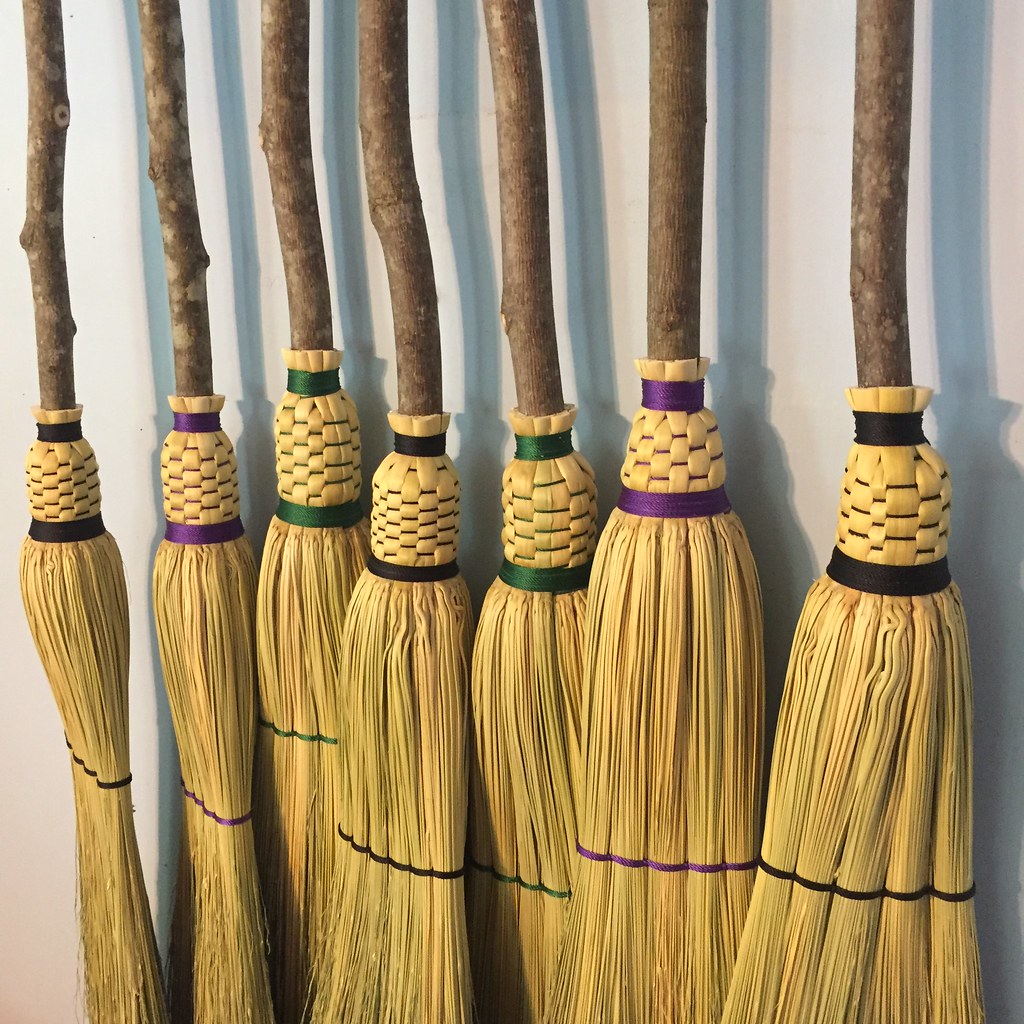The image showcases seven rustic, handmade brooms hanging side by side against a smooth, white wall. Each broom features a handle made from naturally textured and slightly crooked tree branches, adding an old-fashioned, artisanal charm. The straw broom heads are secured to the handles with intricately woven bands that alternate in color. From left to right, the sequence of band colors follows a distinct pattern: black, purple, green, black, green, purple, and black. The black bands occupy the first and last positions as well as the center, while the purple bands are found next to the outer black ones, and green bands are positioned around the central black band. The detailed wrapping of these colored bands not only secures the straw but also adds an artistic touch to the design of each broom.